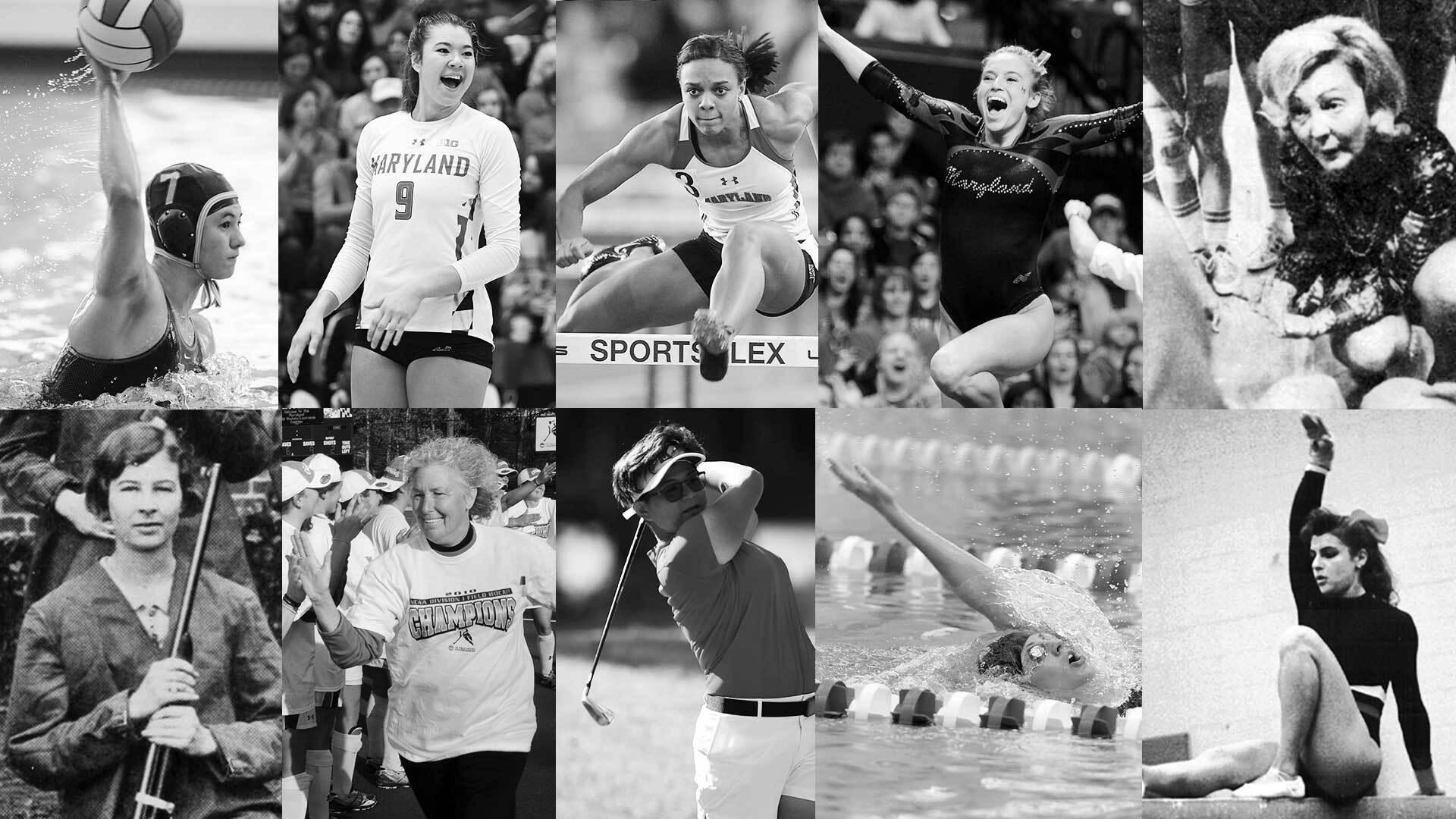This is a detailed composite black and white image featuring 10 vertically aligned photographs of various athletes, organized into two rows of five on top and five on the bottom. 

In the upper left, there is a woman positioned in the water, wearing a tight-fitting helmet labeled with the number seven, holding a volleyball above her head. Next to her is a woman in a jersey with "Maryland" and the number nine, clad in volleyball shorts. The middle photograph showcases an athlete mid-stride, clearly hurdling on a track. Adjacent to this image is a gymnast captured mid-performance. The upper right features an older woman, although her sport is not specified.

The bottom row begins with a man in the lower left firmly grasping the barrel of a rifle in front of him. Next to him, there is a woman in a white t-shirt that reads "Champions," appearing to be running a road race. The subsequent photograph is of a woman golfer mid-swing. Following her is an image of a swimmer in action. Finally, in the lower right corner, there is another gymnast striking a pose. 

Each photograph distinctly highlights different sports and athletes, capturing the diversity and skill across various athletic disciplines.